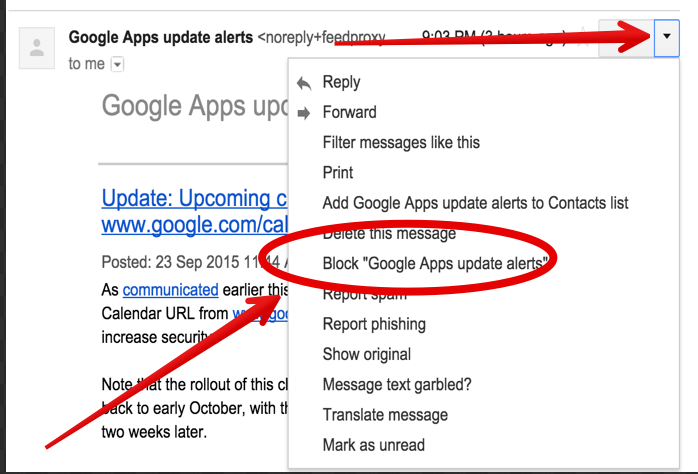The image depicts an interface with a white background displaying multiple notifications related to Google Apps update alerts. It is noted to be 9:03 p.m. In the image, a red arrow prominently points to a drop-down box labeled "Google Apps," indicating updates. Additionally, a white box contains options like "Reply," with a left-pointing arrow, and options for future messages, such as "Print," "Add Google Apps update alerts to contacts list," "Delete this message," "Block," and more. There are red markings, including a circle and an arrow, emphasizing the "Block Google Apps updates alerts" and "Delete this message" options. Other visible options include "Report spam," "Report phishing," "Show original," "Message text garbled?," "Translate message," and "Mark as unread."